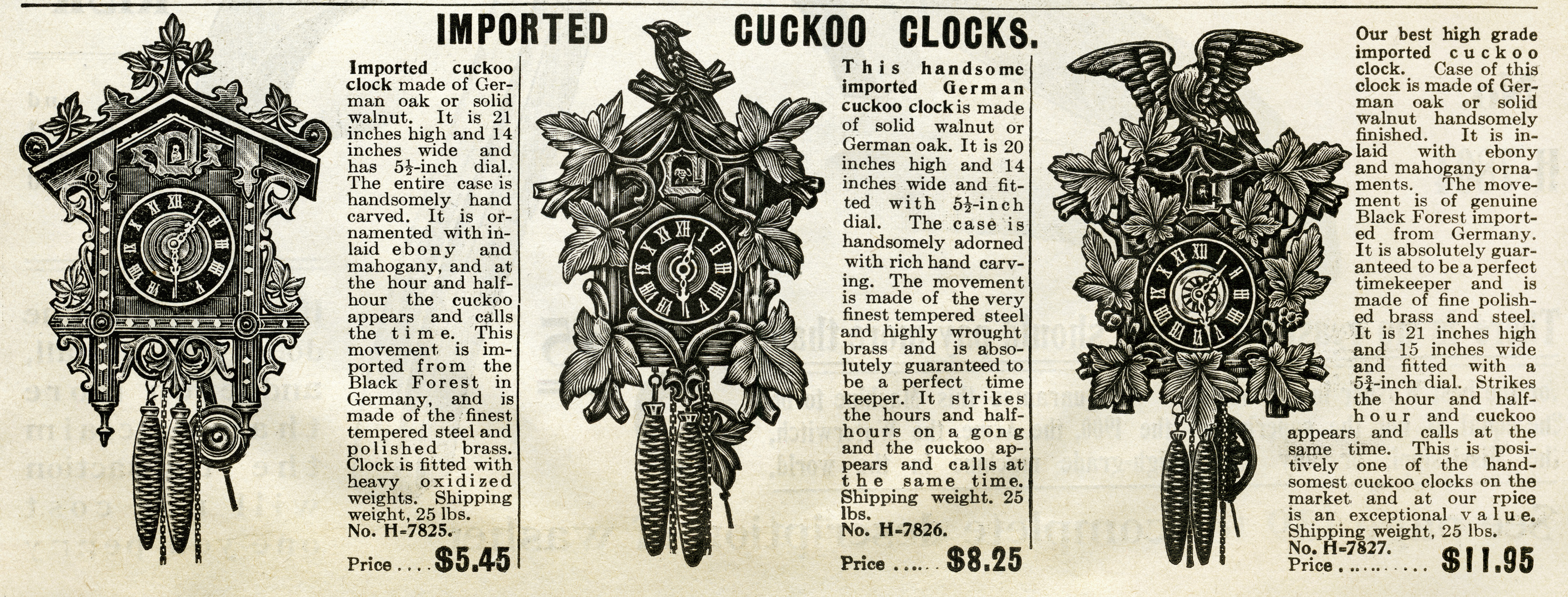The black-and-white image appears to be a clipping from a newspaper, magazine, or catalog, showcasing a vintage advertisement for three imported cuckoo clocks. The ad, which resembles newsprint, features a long rectangular strip divided into three sections, each highlighting a different intricately carved cuckoo clock. Each clock has a unique design with detailed carvings and is accompanied by long descriptive paragraphs and Roman numeral clock faces.

The first clock, priced at $5.45, has a roof adorned with leaves and features two pine cone weights dangling from the bottom. The second clock, priced at $8.25, is topped with a bird and surrounded by leaf carvings, also with two pine cone weights. The most elaborate of the three, priced at $11.95, showcases an eagle with outstretched wings perched on top, surrounded by leaves, and again, with two pine cone weights. Each clock is identified by item numbers H7825, H7826, and H7827, respectively.